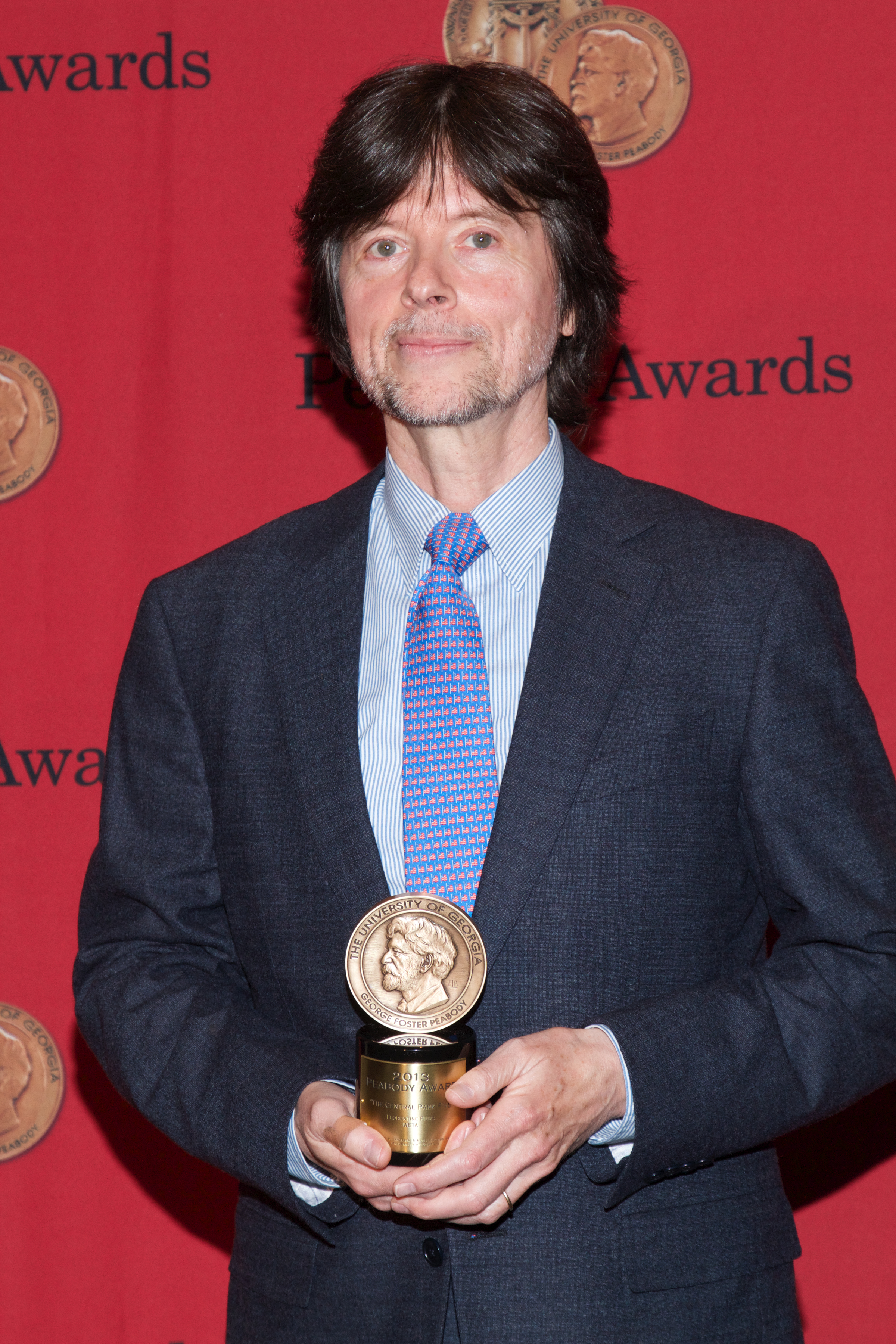The photograph captures documentarian Ken Burns standing in front of a solid red fabric backdrop adorned with two repeating logos. One of the logos, partially obscured by the edges of the image and Ken Burns' head, prominently features the word "AWARDS" in black text. The other logo resembles a medallion, showing a side profile of a man and the words "University of Georgia." Ken Burns, with his short brown hair and stubbly beard, is dressed in a dark blue suit, complemented by a white and blue striped button-up collared shirt, and a blue tie adorned with pink dots. In both his hands, he holds a small round metal trophy, which mirrors the medallion design in the background, featuring a gold plaque that includes the words "University of Georgia" and other details, possibly indicating a film-related award from 2013.